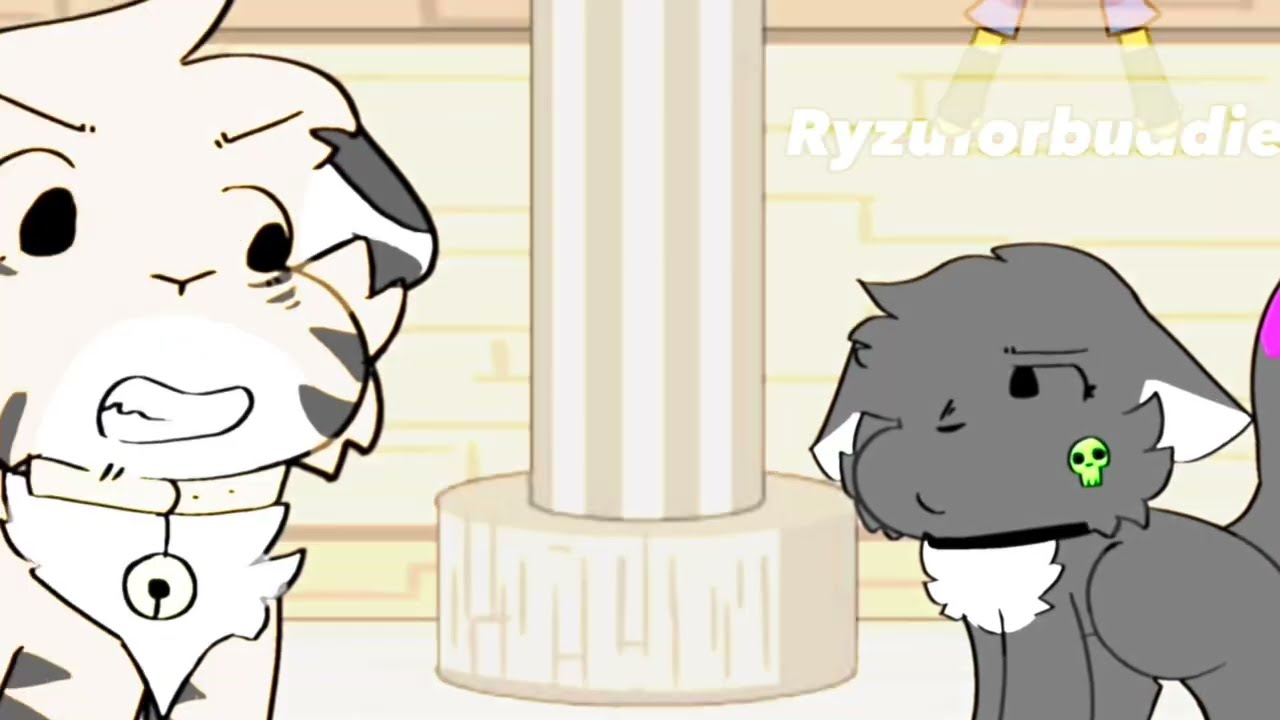This image appears to be a screen grab from an animated cartoon, drawing its style from comic strips. The scene features a museum-like setting with a detailed background that includes a white and beige striped column in the center and a white brick or cement wall. Hanging from the ceiling are illustrated lights that add to the grandeur of the setting.

In the foreground, two cartoon animals, possibly dogs or cats, face each other, hinting at a confrontation. The character on the left has a white body adorned with black tiger-like stripes and dark gray triangles. It has black pupils, a furious expression, and a collar with a bell around its neck. On the right, the character is a dark gray animal with a white patch under its chin, drooping ears, a pink tail tip, and a green skull tattoo on its cheek. This character seems more composed compared to the one on the left.

In the upper right corner of the image, white text reads "Rizno or Buddy," possibly referencing the names of the characters or the title of the cartoon. The detailed artwork and expressions suggest a significant moment or conflict between the two characters in this vividly illustrated scene.